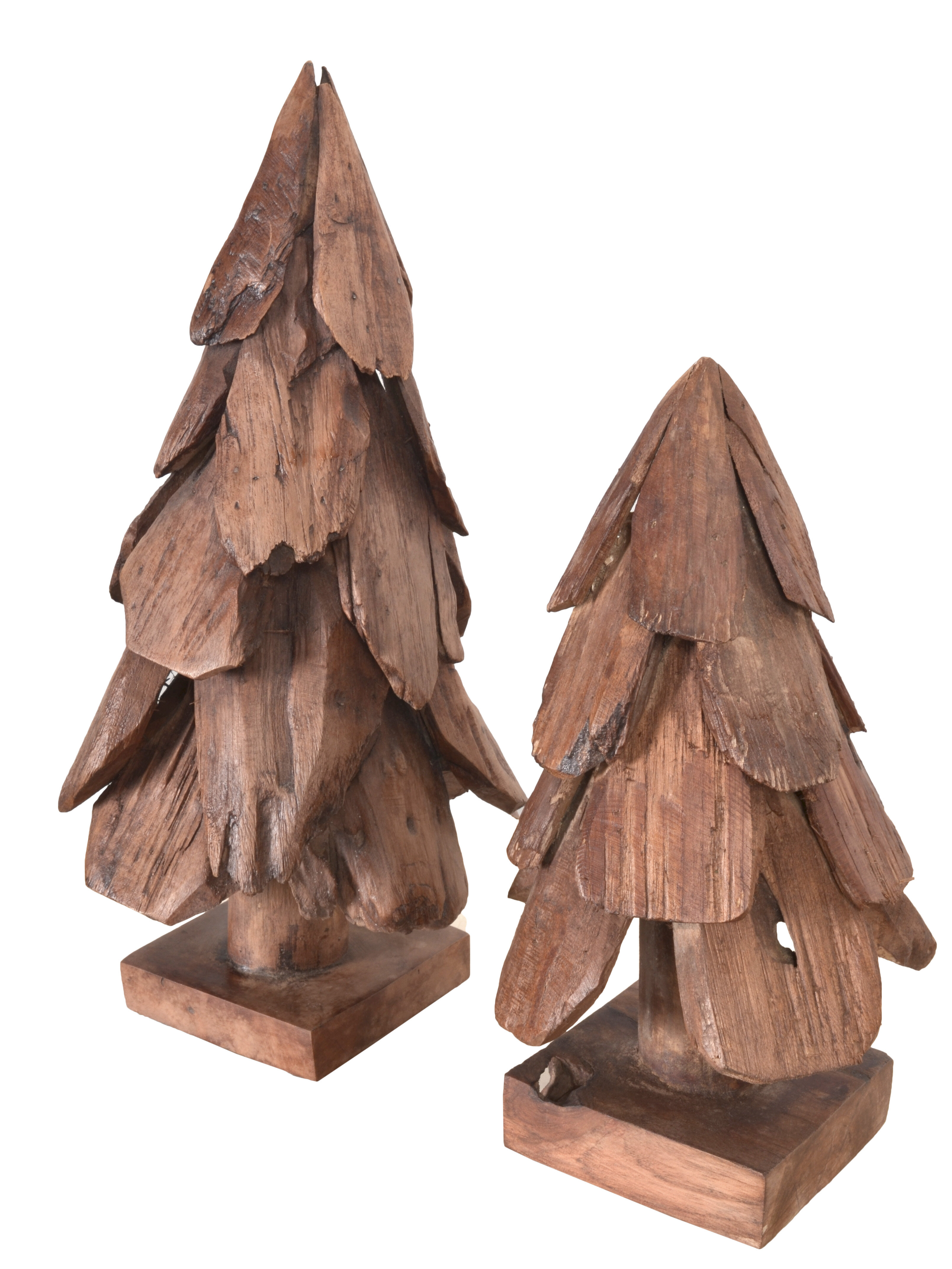This image showcases two carved wooden figurines shaped to resemble abstract pine or Christmas trees. The figures rest on square wooden bases and are positioned against a stark white background, possibly indicating a digital enhancement or light box setup. The taller tree is on the left, while the smaller tree stands to its right. The intricate design includes wood chips meticulously glued together, creating a textured appearance of foliage in varying shades of brown, from light to dark. These handcrafted pieces, which may feature special types of wood such as driftwood, seem to be listed for sale online, highlighting their unique craftsmanship and decorative appeal.